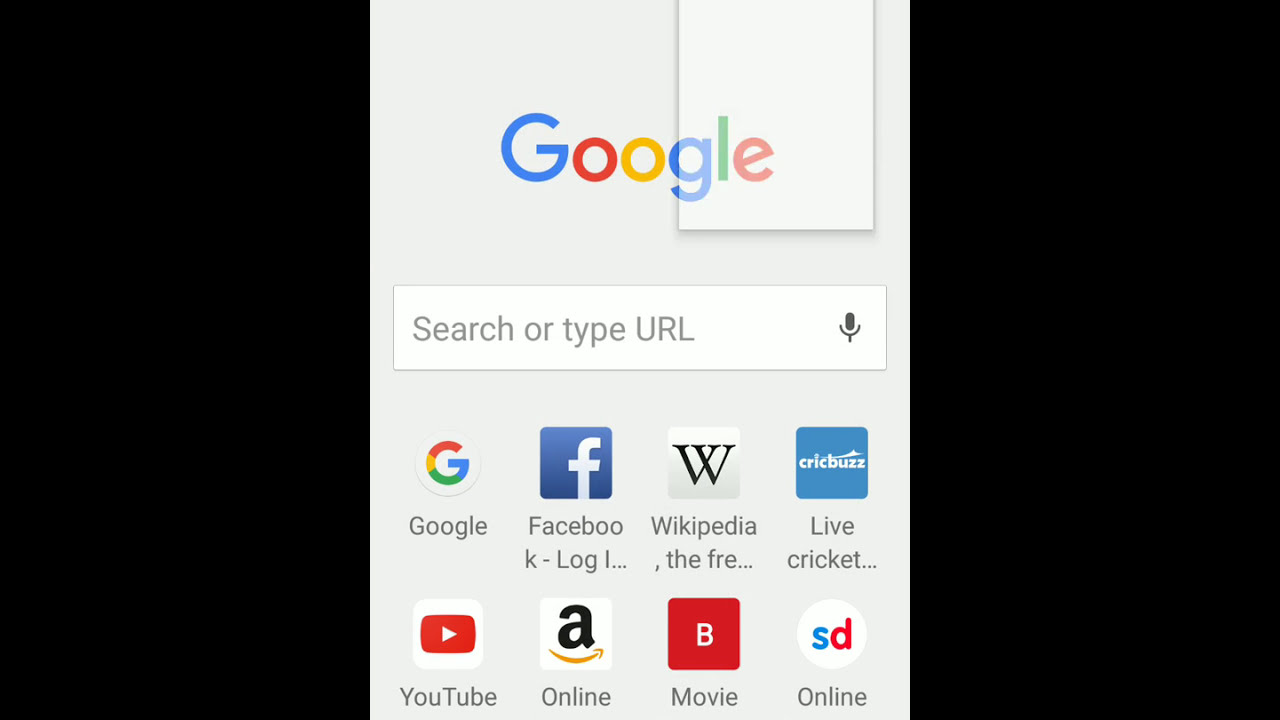This image is a screenshot of a mobile phone screen displaying a web browser. The image itself is framed by two large black vertical rectangles on either side, presumably the borders of the phone. Dominating the center is a white rectangular area. At the very top of this white space, the word “Google” is displayed in a vibrant, multicolored font. Directly beneath this, there is a white search field with the placeholder text "search or type URL" in gray font. At the far right end of this search field is a small black microphone icon.

Below the search field are two rows of app icons. The first row features four icons: 

1. On the far left, a multicolored 'G' icon with the label "Google" underneath.
2. Next to it, a blue square with a white 'F' icon labeled "Facebook."
3. To the right of that, a white square with a black 'W' icon representing "Wikipedia."
4. Finally, a blue square with the text "Cricbuzz" in white font, followed by the subtext "Live Cricket."

The second row contains a single app icon:

1. On the far left, a white box containing a red box with a white play arrow inside it, labeled "YouTube."